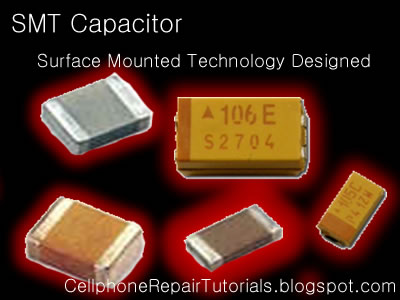The image features a black background with white text in the upper left corner that reads "SMT Capacitor." Centered below it, in smaller font, is the phrase "Surface Mounted Technology Designed." At the bottom of the image, the text "CellPhoneRepairTutorials.blogspot.com" is displayed. The main focus of the image is five SMT capacitors, each surrounded by a red glow. 

- The top left capacitor is a small, rectangular component with two white edges and a gray center. 
- In the middle is a larger, yellow capacitor labeled "106E S2704."
- Below it is a longer, thinner capacitor. 
- To the right, there is another yellow capacitor.
- To the left, there's a capacitor that is white and brown.

All capacitors in the image feature silver-colored ends. The capacitors display a mix of silver, gold, yellow, and brown shades, and the background remains completely black, emphasizing the components and their descriptions.